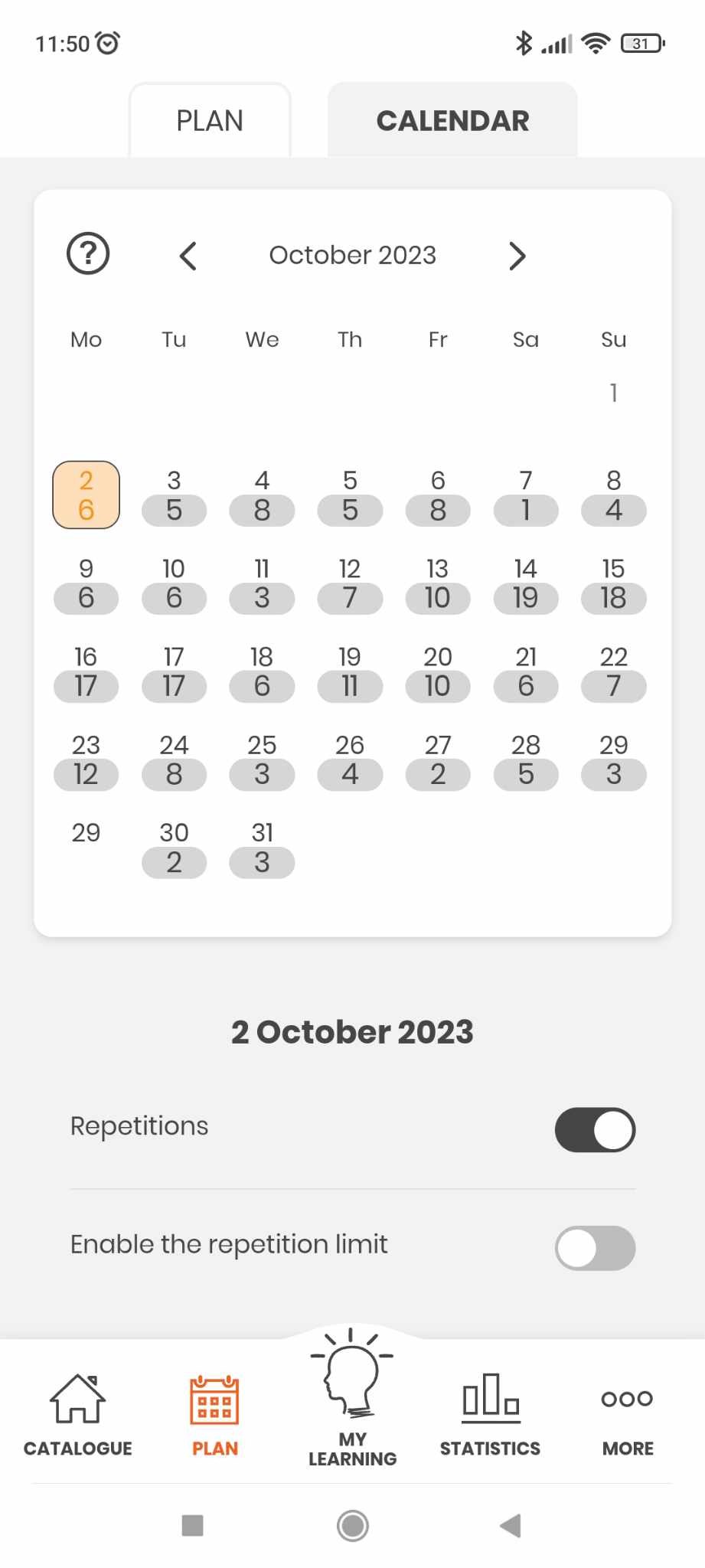Here's a detailed and cleaned-up caption for the provided image:

---

The screenshot displays a tablet interface of a time management and planning application, showcasing its "Calendar" tab for October 2023. The user interface is simplistic and intuitive, featuring a white background contrasted with black block print text.

In the upper left corner, there are two tabs labeled "Plan" and "Calendar." The "Plan" tab, while visible, is not currently selected; it has a plain white background. Dominating the screen is the active "Calendar" tab, highlighted with a pale blue background. 

At the center of the "Calendar" tab is the October 2023 monthly view. Each day of the month is marked with an oval blue bubble displaying a number beneath the date. These numbers vary and appear to represent counts of specific activities or repetitions logged by the user.

Immediately below the calendar view, the date "2 October 2023" is highlighted with additional settings exposed. There is a label "repetitions" accompanied by a slider button set to "On," which has a black background. Following this, there is another option labeled "enable repetition limit," which features a slider button currently set to "Off," indicated by a slightly darker blue shade on a pale blue background.

At the bottom of the screen, a navigation bar displays five options, each accompanied by an icon: "Catalog" (depicted by a house icon), "Plan" (calendar icon), "My Learning" (brain with rays), "Statistics" (graph icon), and "More" (ellipsis icon).

Reading the numbers below the dates from left to right, starting from Monday, October 2nd, the numbers listed are: 6, 5, 8, 1, 4, 6, 6, 3, 7, 10, 19, 18, 17, 17, 6, 11, 10, etc. While their exact purpose is unclear to the observer, they likely represent the user's logged activities or repetitions for each respective day.

---

This caption provides a comprehensive and clear description of the screenshot, detailing each element and its potential function within the app.